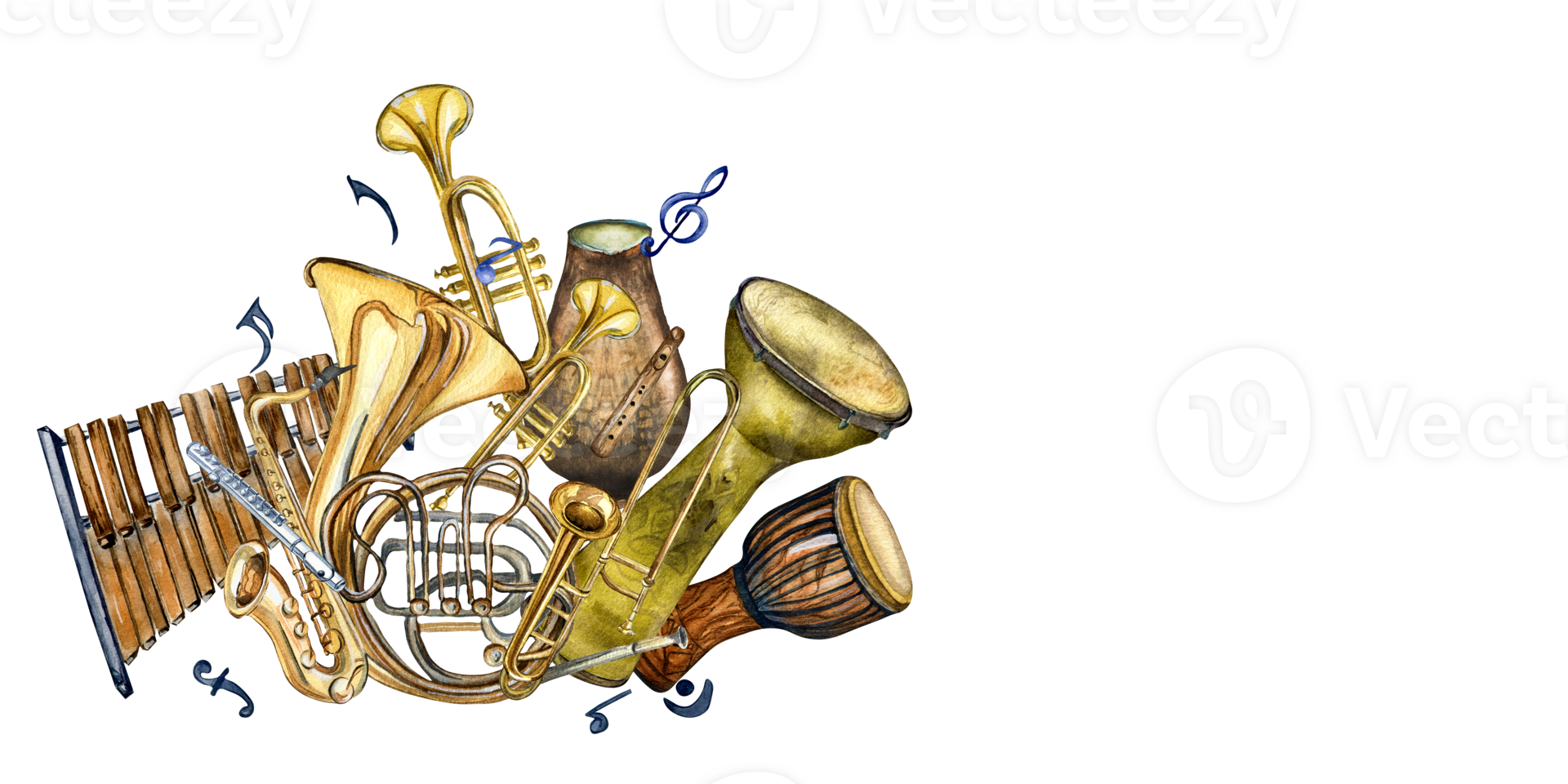This colored drawing is an elaborate and dynamic sketch of various musical instruments, seemingly alive and playing music in unison. From left to right, the image showcases a wind flute or windpipe, a saxophone, a trumpet, and a tuba or French horn. Several vase-shaped drums with skins on top are positioned in different areas, including three bongo drums near the bottom right of the image. Additional instruments such as a xylophone, a trombone, and perhaps a clarinet contribute to the rich assortment. Musical notes in blue hues surround and pop out of the instruments, enhancing the illusion that they are playing music on their own. The instruments appear animated, brimming with life, and together they form an enchanting, harmonious band. Amidst this lively collage of instruments and notes, a watermark reading “Vek Tisi” is subtly visible. The overall color palette consists of neutral, metallic tones, giving the drawing a cohesive and rich texture.